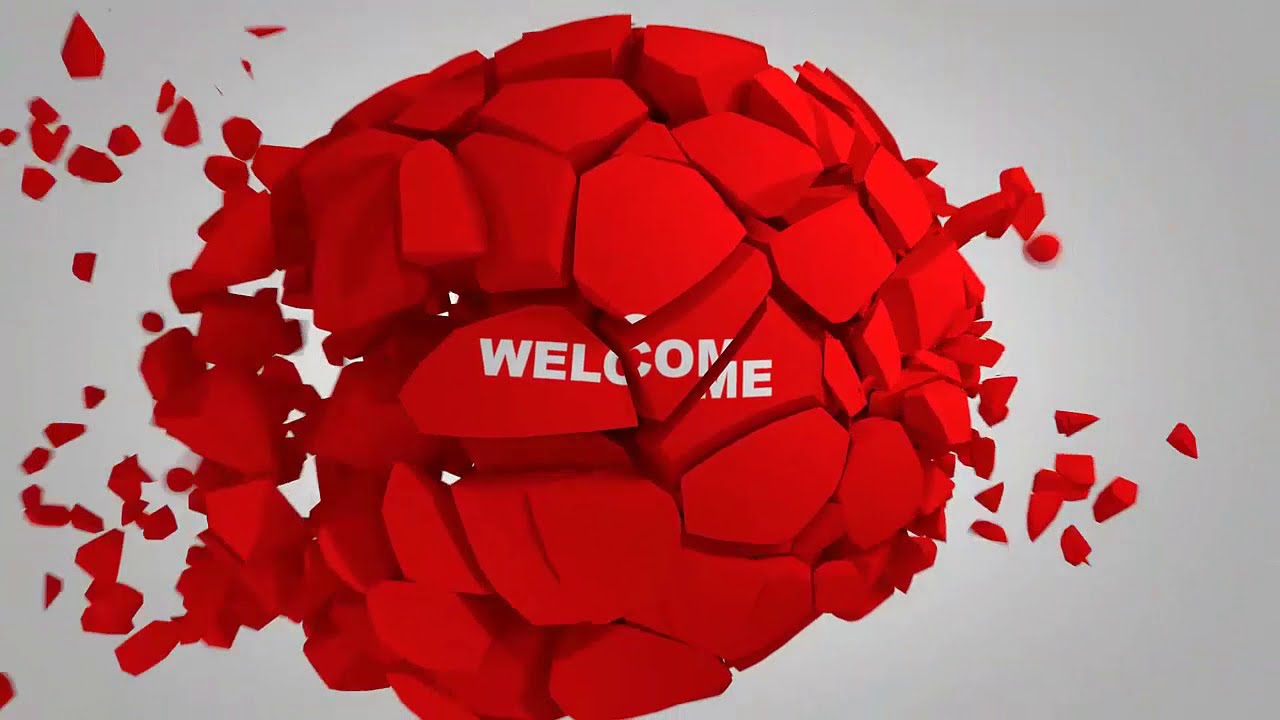The image depicts a graphics-designed spherical structure, seemingly once a solid ball, now fragmented into multiple pieces. It bears the word "welcome" in gray or possibly white letters. The spherical object appears to have experienced significant damage, most notably on the left side, where larger and more numerous chunks are dispersing. In contrast, smaller fragments trail off to the right, suggesting the sphere's gradual disintegration. The background is a solid gray with a subtle gradient, lightest at the center behind the sphere and darkening towards the edges, giving the impression of a light source. Larger shards, still retaining some form of the sphere, are interspersed with jagged shapes like hexagons, squares, and triangles, scattered predominantly around the central structure. The breaking of the sphere, possibly rendered in a clay-like texture but computer-generated, suggests dynamic motion, as fragments fly off and descend away from the core, evoking the sense of a still-moment of an explosion or a bounce.